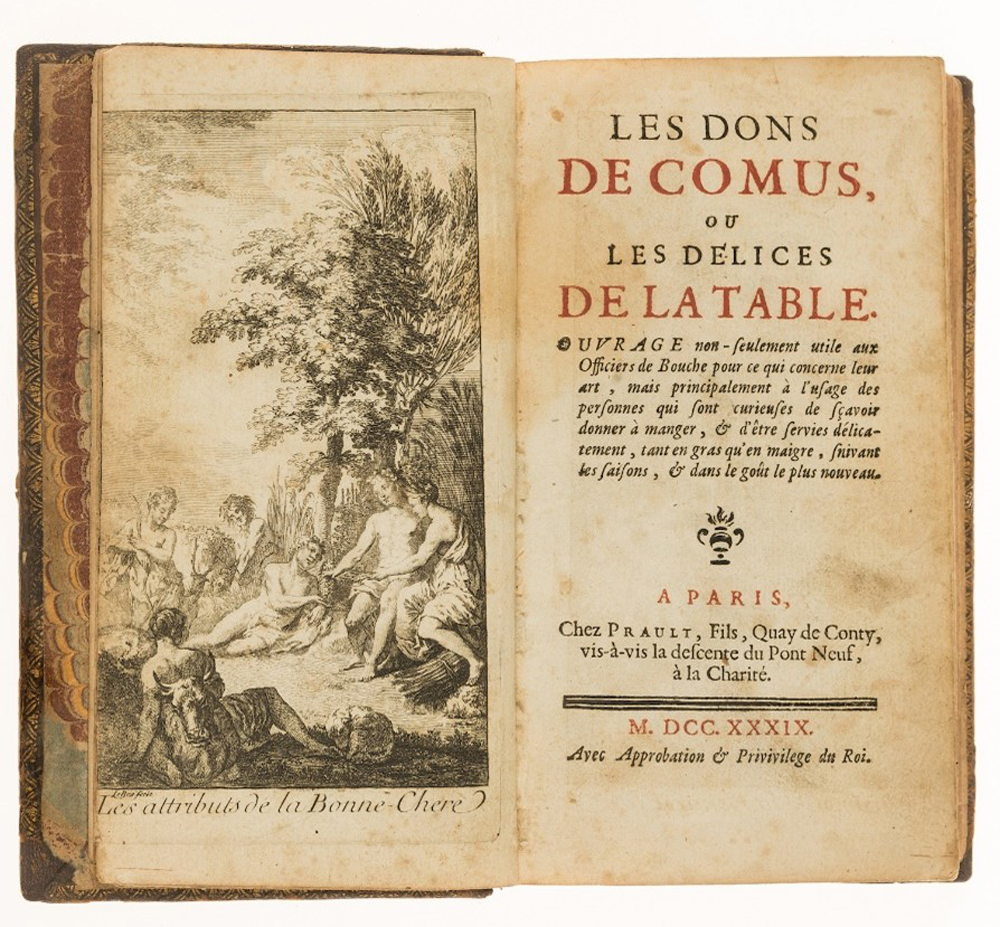This image depicts an open, hardback book with aged, yellowish-brown sepia-toned pages that have marbled edges and finger indentations for easy turning. The left page features a black-and-white, rectangular illustration in portrait orientation, showing five or six people dressed in robes or togas, with some partially nude from the chest up, reclining affectionately under a tree. The scene appears nostalgic and historical, suggesting an earlier time period. On the right page, written in French, is text predominantly in black with some red accents. The text includes the title "Les Dons des Comus, Les Délices de la Table," mentions "à Paris," and dates to "m.dcc.xxxix" (1739).